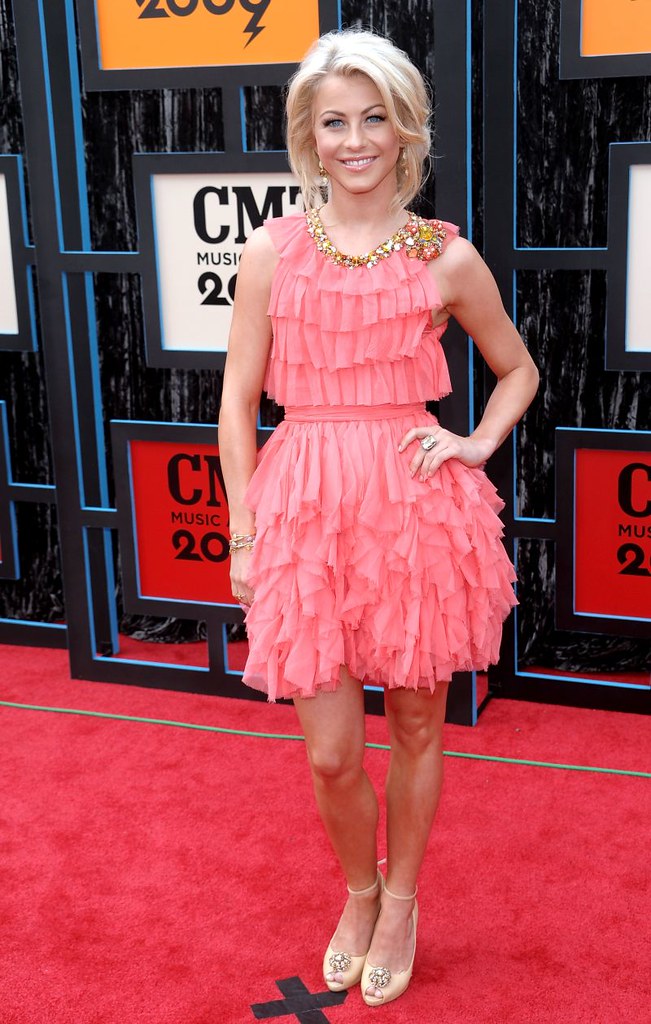In this detailed photograph, a woman is elegantly posing on a red carpet, marked with a black X where she is slightly behind. She dons a ruffled, sleeveless salmon pink dress that cuts off at the shoulders, adorned with a decorative gold trim around the collar, and the outfit features multiple rows of ruffles both at the top and above the knee-length hem. Her light brown, almost blonde hair cascades down to her shoulders, and she wears cream-colored shoes. The woman is well made up, smiling directly at the camera with one hand placed confidently on her hip, and a ring visible on one finger. The background features three doorframe-like cutouts adorned with CMT Music signs, suggesting a music awards event. The dark background contrasts with the well-lit carpet area, highlighting the event's likely daytime setting.